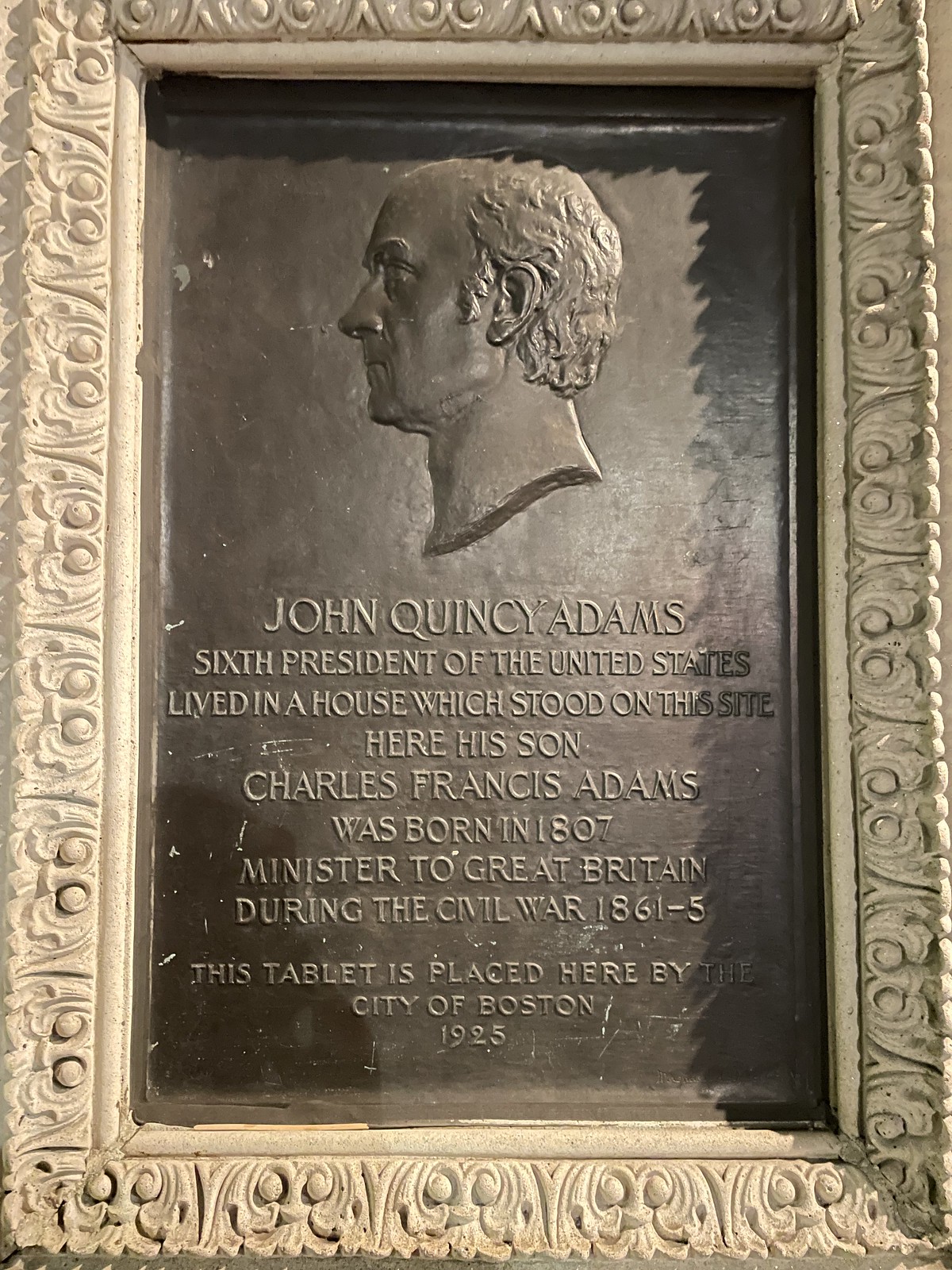The image depicts a framed plaque with a highly intricate and decorative design, likely crafted from marble or concrete. Although the once-white frame has begun to discolor with age, its elaborate carvings remain striking. The plaque itself is silver or gray and features a profile view of a bald-headed man with hair around the sides, identified as John Quincy Adams. The detailed inscription on the plaque reads: "John Quincy Adams, sixth president of the United States, lived in a house which stood on this site. Here his son, Charles Francis Adams, was born in 1807, minister to Great Britain during the Civil War (1861-1865). This tablet is placed here by the city of Boston, 1925."